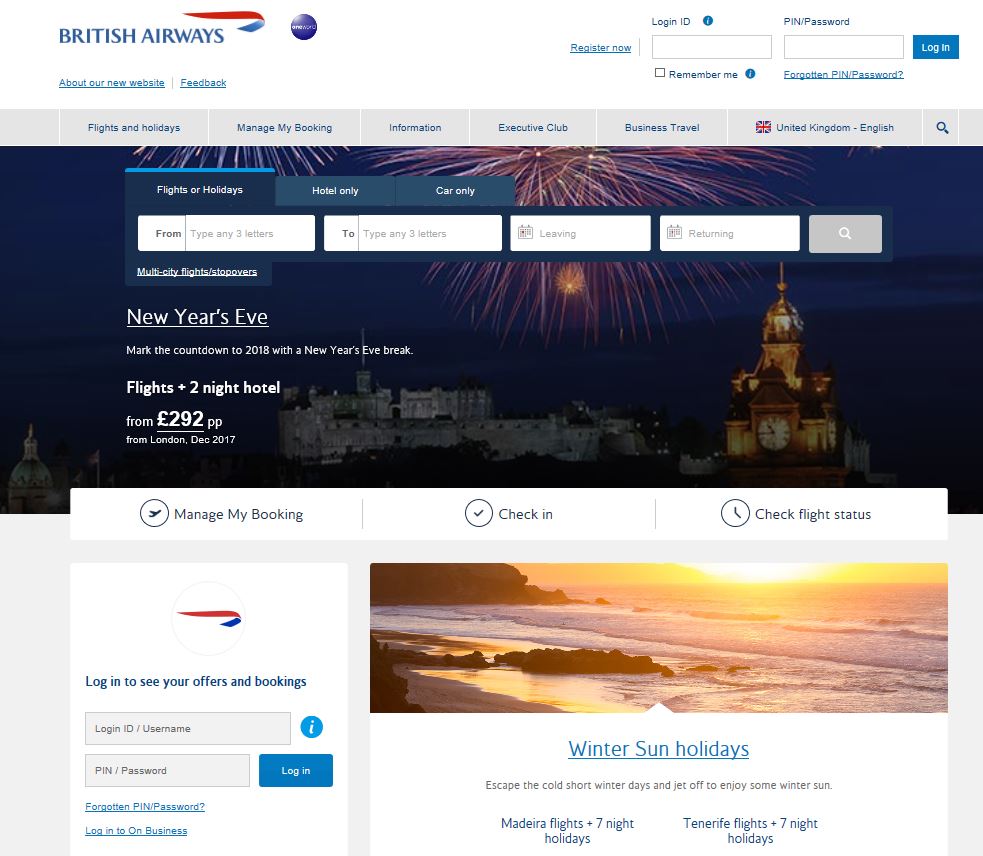This image showcases the British Airways website. In the top left corner, the prominent British Airways logo is displayed in blue text. Below the logo are two clickable links titled "About our new website" and "Feedback". To the right, users have the option to register or log in using their ID and password. 

A gray navigation bar spans the width of the page below, featuring blue links with various options: "Flights and Holidays", "Manage My Booking", "Information", "Executive Club", "Business Travel", and "United Kingdom English". Directly underneath this bar, there is a search area where users can enter their preferences for "Flights or Holidays", "Hotel only", and "Car only".

Further down, an advertisement promotes New Year's Eve travel deals with the tagline, "Mark the countdown to 2018 with a New Year's Eve break. Flights plus a two-night hotel from £292 from London, December 2017." 

Below the advertisement, three specific options are provided: "Manage My Booking", "Check-in", and "Check Flight Status". 

At the bottom left of the page, a prompt encourages users to log in to view their offers and bookings. To the right, there is an image of a beach, accompanied by the text "Warm winter sun holidays" in blue.